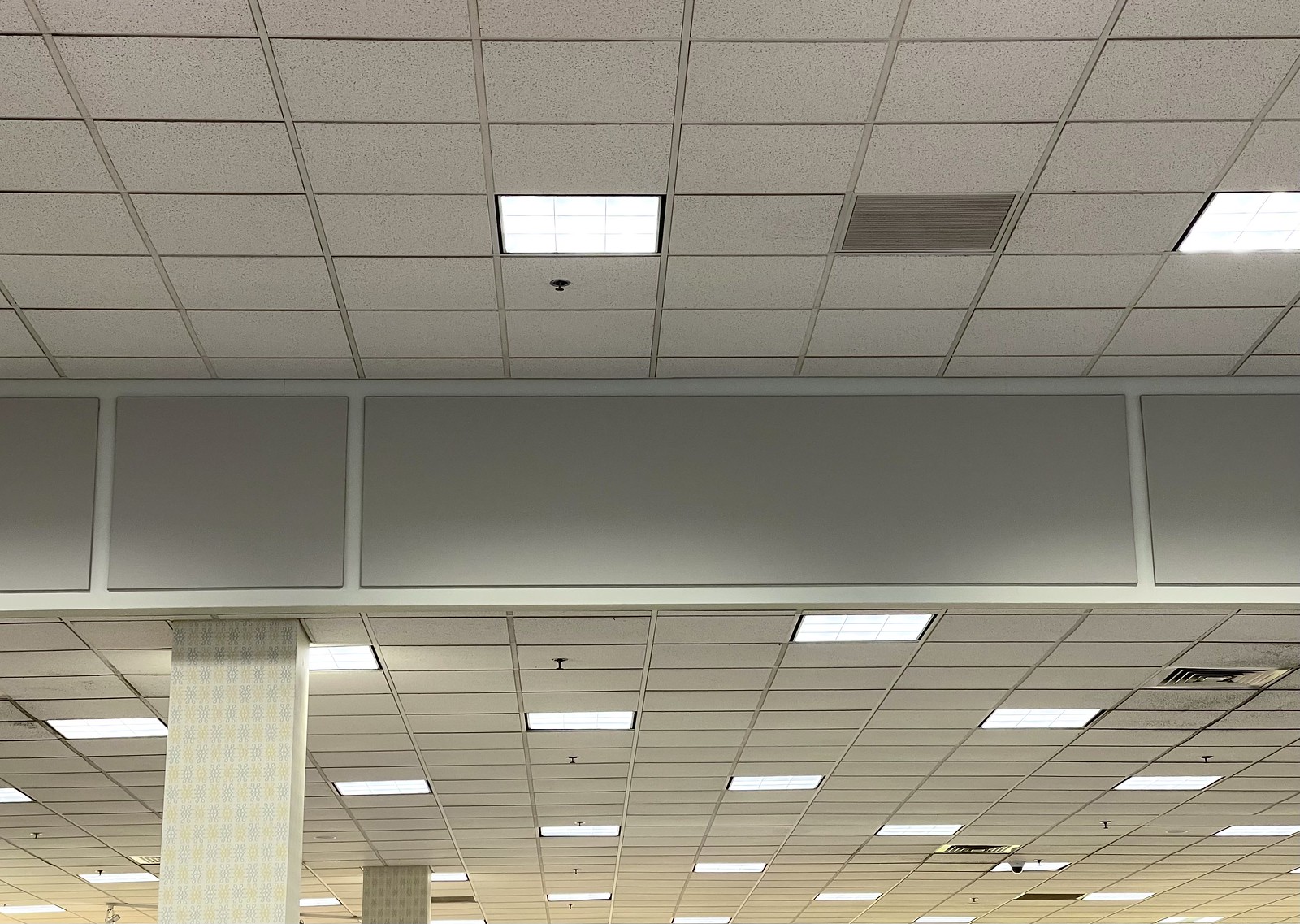The photograph captures the detailed ceiling of a large office building, designed with cost-effective materials typically found in call centers or inexpensive office structures. The image is moderately wider than it is tall and features a grid-like pattern of off-white, rectangular ceiling tiles. These tiles are interspersed with evenly spaced, bright, white square lights and occasional gray vents. Fire sprinklers are also scattered across the entire ceiling, contributing to the orderly yet functional aesthetic.

Prominent in the composition are two structural pillars: one located about six tiles from the left edge of the photo and another around twelve tiles from the first. These pillars support the ceiling and add a slight variance to the otherwise uniform pattern. The ceiling is divided horizontally by a gray tiled border that distinguishes a lower section from an upper section. The lower section features the same rectangular tiles in perspective with the lights and vents, descending towards the bottom edge of the photo. The top section continues the pattern, ascending towards the top edge.

The image highlights the practicality and convenience of such ceiling designs, which facilitate easy access for repairs and installations. The overall lighting is bright, illuminating the room effectively, though only the ceiling and its components are visible in this meticulously arranged shot.